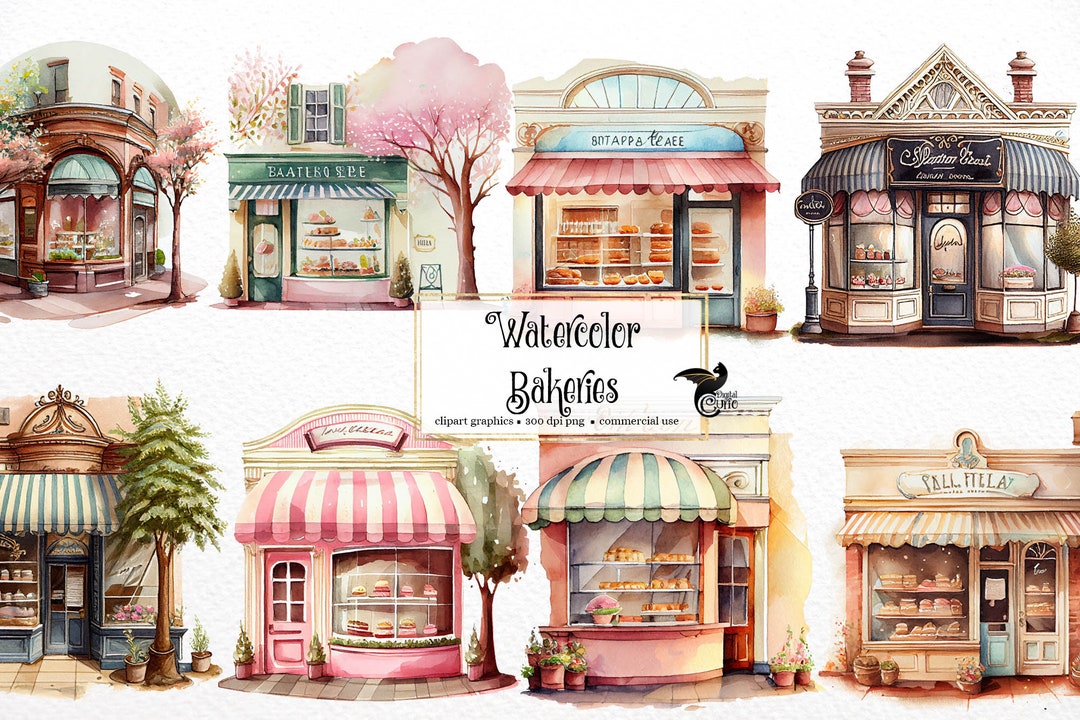This watercolor painting, titled "Watercolor Bakeries," features eight distinct bakeries arranged around a central white rectangle with the label "Watercolor Bakeries" written in black type. The bakeries are meticulously illustrated, with four positioned above and four below the central text. Each bakery showcases a front facade with glass windows or sets of windows, offering glimpses of various baked goods such as cakes, pies, muffins, pastries, and fruits displayed on shelves. Several bakeries feature uniquely designed awnings, with alternating vertical stripes in either green and white or pink and white, adding to their charm. The architectural styles range from sophisticated Victorian designs to more homely, mom-and-pop exteriors, complete with clean, plain doors and individual logos. The artwork also includes decorative elements like pink and green flowers and lush trees surrounding the buildings, enhancing the quaint, picturesque atmosphere of the scene.